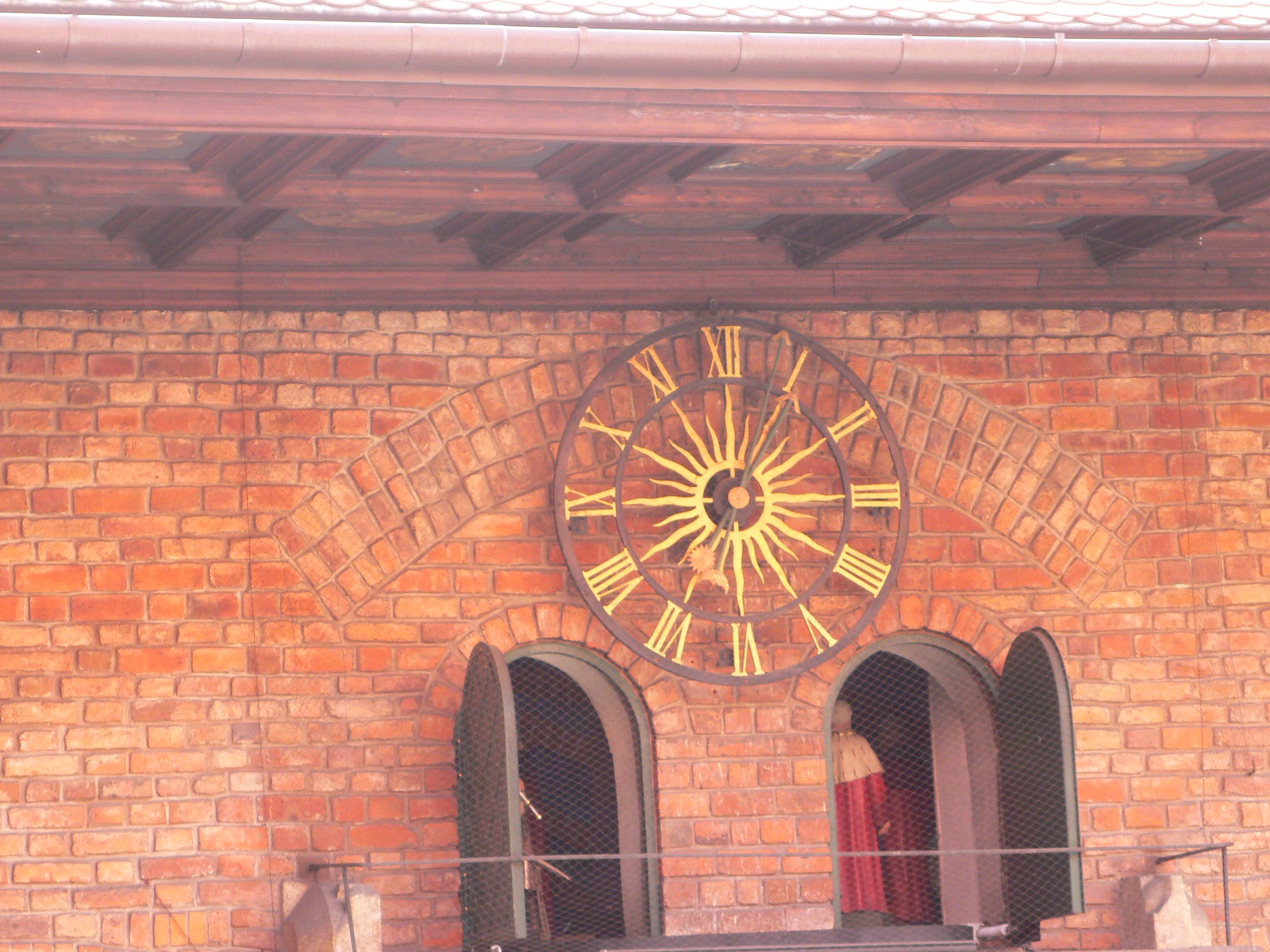This photograph captures the upper section of a red, brown, and orange brick building. Central to the image is a large, ornate clock made of brown-coated steel. The clock features golden Roman numerals encircling a central sunburst design with wavy lines radiating outward, and has black hands adorned with crescent moon and sun motifs. The clock is mounted beneath a timber-framed roof that projects outward, adding a rustic touch with its color mosaic. Flanking the clock are two arch-shaped windows lined with mesh, housing figurines dressed in long red robes with light brown accents around the neck and white fur-trimmed capes. These figures stand behind dark chocolate brown doors, and the mesh likely serves to prevent birds from entering. At the top of the photograph, wooden frames part of the roof structure are visible, contributing to the overall architectural detail.